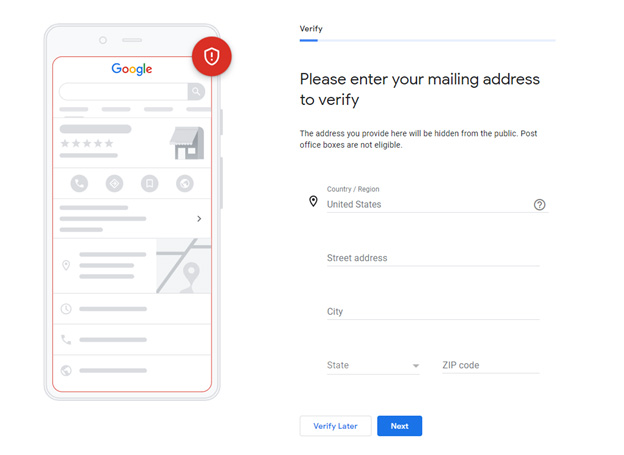The image showcases two elements: a cell phone on the left and an open webpage displayed on the phone to the right. The cell phone's screen features a clean white background with the word "Google" prominently displayed at the top in its distinctive multicolored letters. Below the Google logo, a red circular line borders a shield icon containing an exclamation mark, indicating attention or caution.

Proceeding below, there is a section labeled "Verify," highlighted by a blue line. The text instructs the user to "Please enter your mailing address to verify." It clarifies that the address provided will be hidden from the public and that post office boxes are not acceptable. The form fields request information for "Country/Region," preset to "United States," followed by fields for "Street Address," "City," "State," and "ZIP Code."

At the bottom of the webpage, there are two interactive options: a white button labeled "Verify Later" and a blue button labeled "Next."